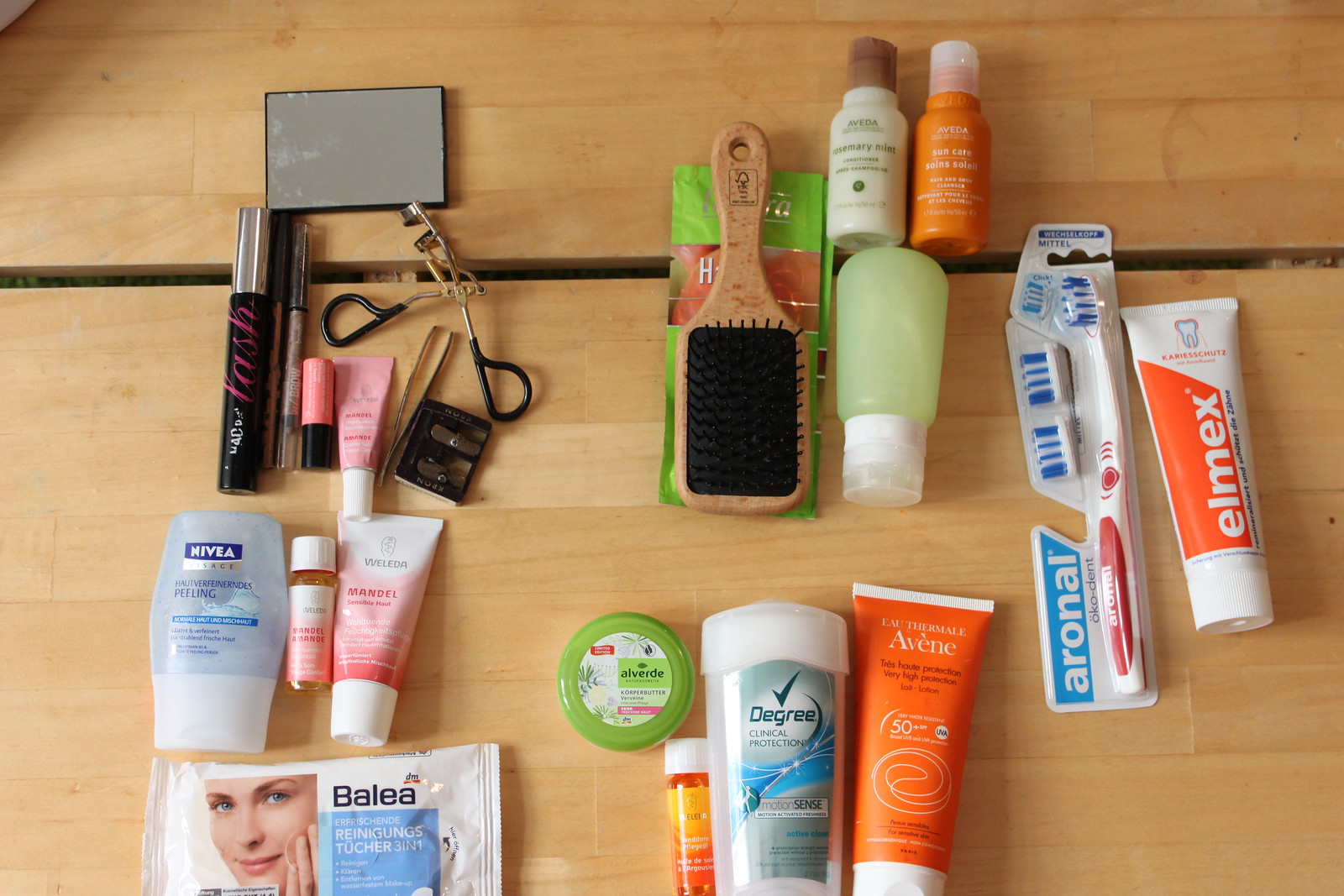A well-used, light-colored table with slightly dingy and stained surfaces, featuring a middle section designed to accommodate an extra leaf piece for expansion. The table is adorned with an assortment of beauty items, each meticulously arranged. Among them is a black and pink mascara with a silver lid, accompanied by a small, rectangular mirror encased in black plastic. An open eyelash curler with black handles lies nearby, next to a pencil sharpener. A pink and white labeled tube of lotion stands close to a clear, round Nivea bottle. The spread also includes a Degree Clinical Protection deodorant, makeup wipes in a white and blue package displaying a woman's face, and a sealed red toothbrush with several additional brush heads. Completing the collection is a wooden paddle brush with a black base, showcasing the diverse range of beauty and personal care products on the table.